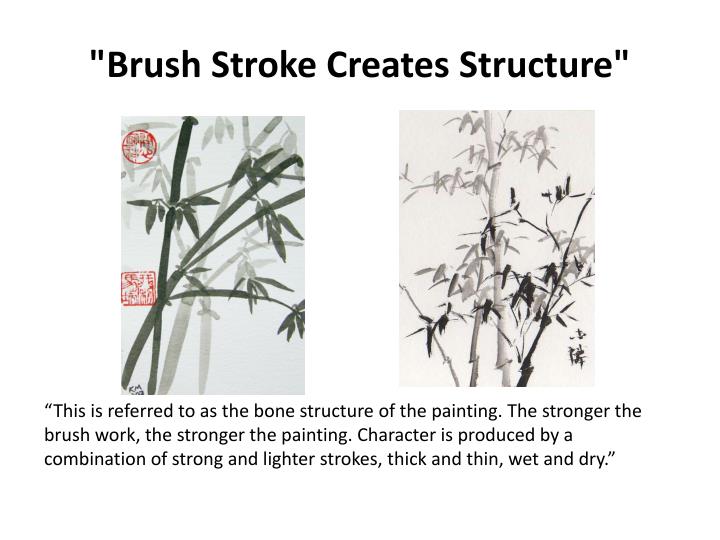The image depicts a presentation slide from a how-to book on traditional Japanese painting, focused on the concept of "Brush Stroke Creates Structure." Two side-by-side photographs of paintings showcase bamboo plants, each depicted with varying brush techniques. The painting on the left features bold green brush strokes with a red stamp and Chinese characters in the top left corner, and an additional square stamp beneath it. It illustrates bamboo reaching from the bottom left to the top right. The painting on the right, akin in composition, utilizes shades of black and portrays the bamboo growing from the bottom center towards both the top center and the sides. It includes a signature in the bottom right corner. Both paintings are set against a white background. Below these images, the quoted text reads: "This is referred to as the bone structure of the painting. The stronger the brushwork, the stronger the painting. Character is produced by a combination of strong and lighter strokes, thick and thin, wet and dry." This emphasizes the significance of brush technique in creating the structural integrity and expressive quality of the paintings.